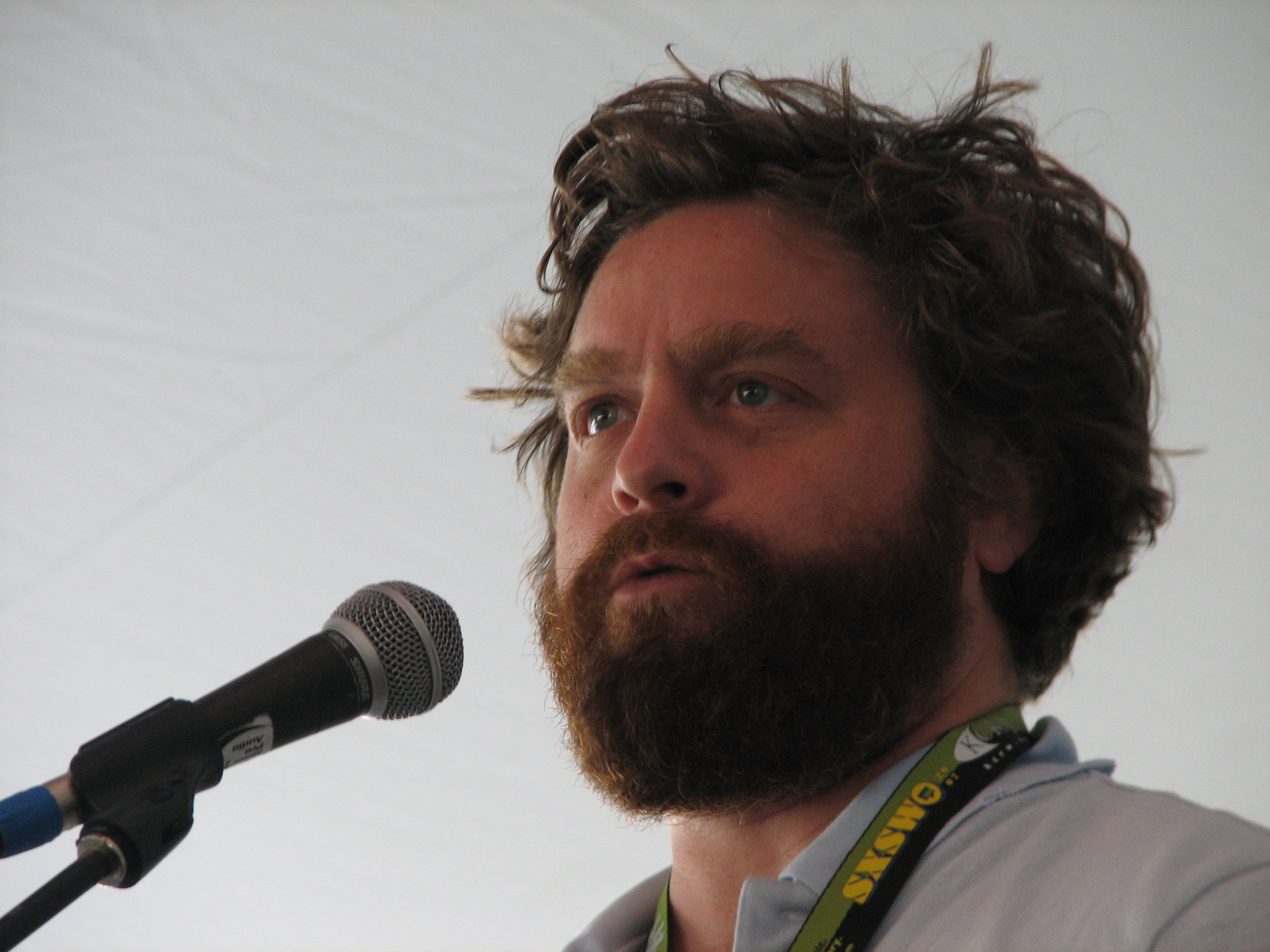The image is a detailed headshot of a man, resembling Zach Galifianakis, who appears to be either talking or performing with a microphone. The man is positioned slightly angled towards the left, with his head centered in the frame. He has brown, tousled hair, blue eyes, and a stern expression accented by furrowed brows. His facial hair includes bushy eyebrows, a mustache, and a very bushy beard. He wears a light blue collared polo shirt and a green lanyard with yellow lettering, reading "SXSW," indicating the South by Southwest event. His skin has a reddish-pink hue, suggesting a slight sunburn. The microphone and its stand are visible at the bottom left of the image, characterized by shades of gray, black, and a hint of blue. The background is a simple white, possibly a sheet, emphasizing the subjects in the foreground. The overall setting suggests a formal occasion, likely a speech or Q&A session at South by Southwest.